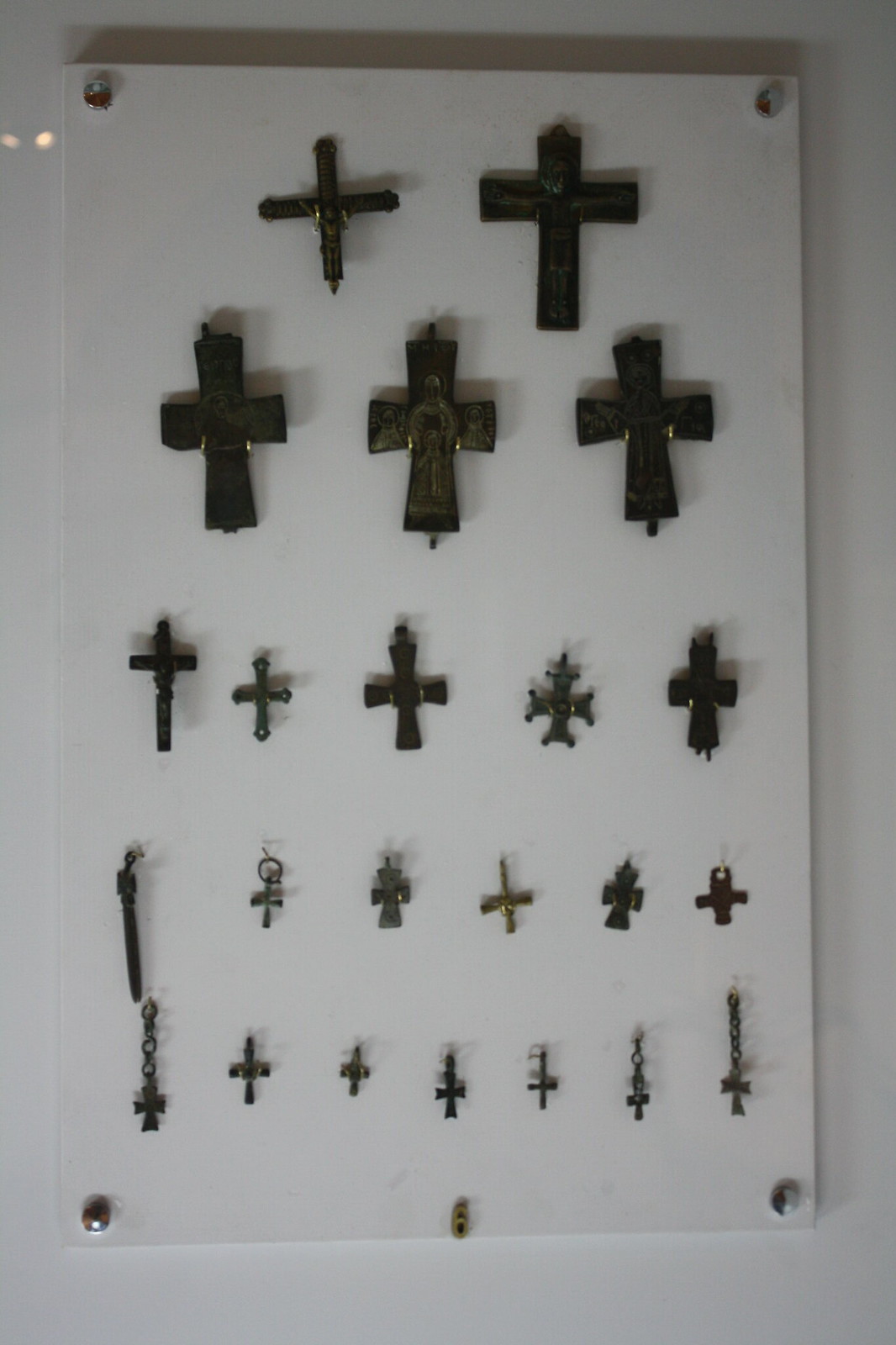This color photograph, taken in portrait orientation, showcases a white wall on which a white board has been firmly screwed into place. The board, which features visible drill holes in each corner secured with screws, supports an arrangement of black crosses. These crosses, varying in size and style, are affixed with small pins and tacks. 

The display is organized into five distinct rows: the first row contains two large crosses, the second row features three crosses of similar size, and the third row holds five slightly smaller crosses. The fourth row displays six even smaller crosses, and the final row comprises seven of the smallest crosses in the arrangement. Some of the lower crosses are adorned with little chains, suggesting they might be fashioned to resemble necklaces.

The crosses themselves exhibit a variety of designs, from simple two-stick constructions to more intricate shapes, potentially including fleur-de-lis patterns. The entire setup, with its lack of vibrant colors, is highlighted by two small pin lights positioned along the left side of the wall, casting a focused illumination on the display.